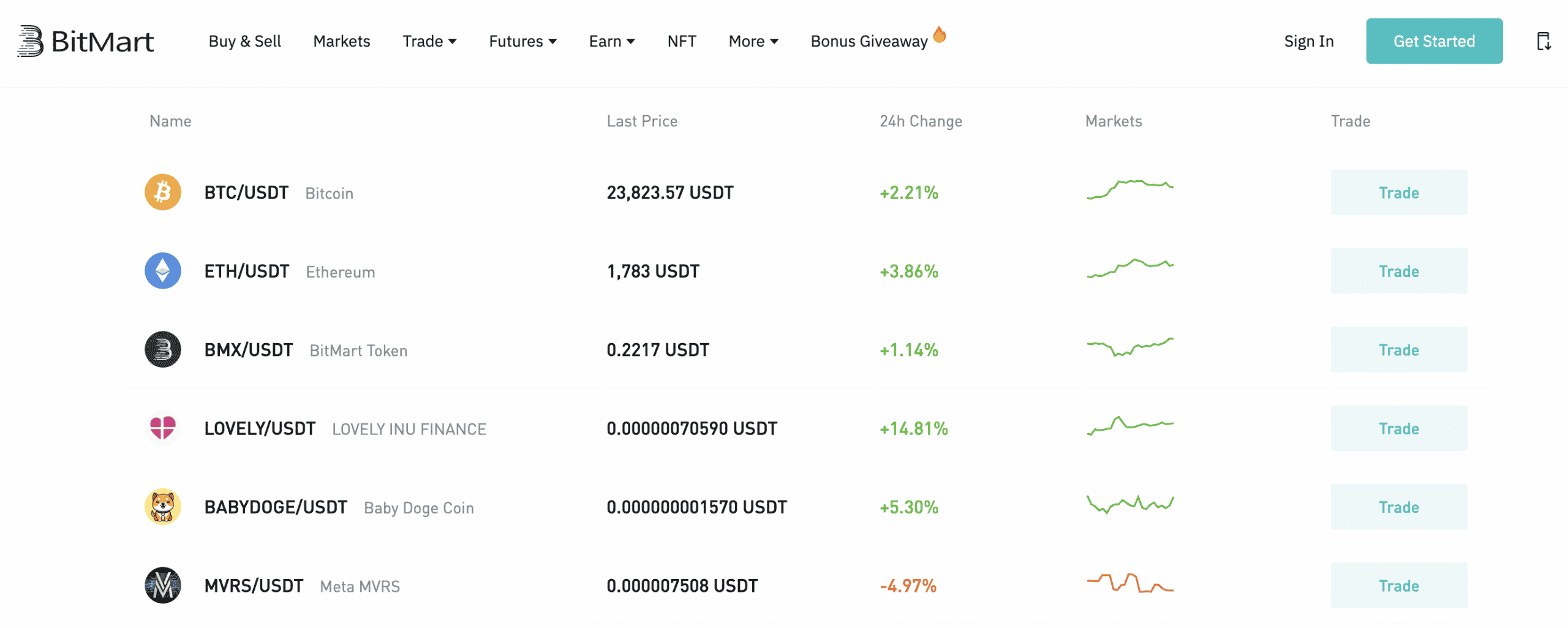The image displays a detailed screenshot of the BitMart Bitcoin exchange web page. The top section of the page has a navigation bar with various options in black text, including "Buy and Sell," "Markets," "Trade," "Futures," "Earn," "NFT," "More," "Bonus," "Giveaway," and an additional icon on the far right whose function is unclear. To the right of these options, there are two primary action items: a "Sign In" button in black text and a "Get Started" button featuring a teal background with white text.

Beneath the navigation bar, the main body of the page presents a comprehensive list of cryptocurrency pairs. These pairs are formatted as combinations of base and quote currencies, such as BTC/USDT (Bitcoin to USD Tether), ETH/USDT (Ethereum to USD Tether), and various others including BMX/USDT, LOVELY/USDT, BabyDoge/USDT, and MVRS/USDT. Each cryptocurrency pair row includes several columns: 

1. **Last Price**: Displays the most recent trading price for each pair.
2. **24H Change**: Indicates the percentage change in price over the last 24 hours.
3. **Market Chart**: A small line graph representing recent price movements.
4. **Trade Button**: A clickable button that allows users to initiate a trade for the selected cryptocurrency pair.

The structured and detailed layout provides users with essential trading information and direct access to trading functionalities.